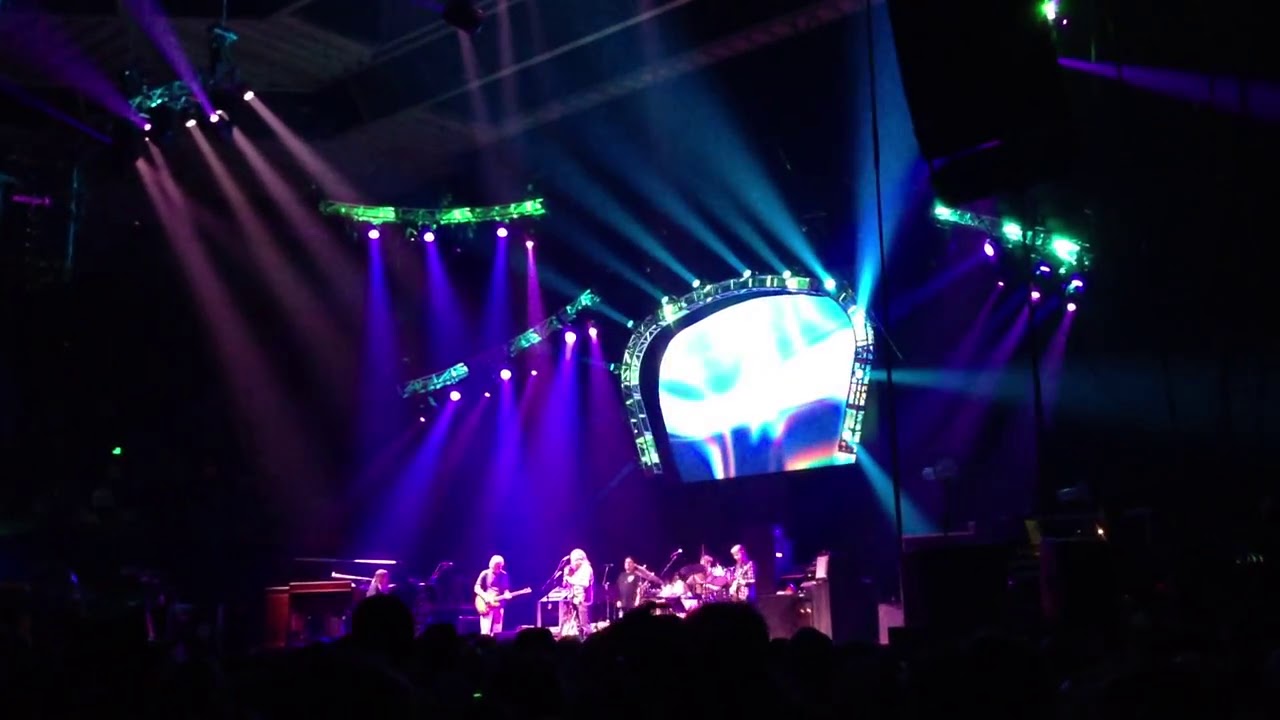This indoor concert image captures the vibrant atmosphere of a packed audience, silhouetted by the dark, rounded heads at the bottom foreground, indicating the photographer is amidst the crowd. The stage, bathed in shades of blues, purples, and magenta lighting, showcases a dynamic setup with various musicians: a guitarist to the left, a keyboardist or pianist to the right, a bass guitarist positioned centrally, accompanied by two additional guitarists and a drummer in the background. Floodlights beam down from above, with some illuminating the stage while others shine upwards and outwards towards the walls and audience. Dominating the background is a large, reflective, horseshoe-shaped screen with lights surrounding it, creating a captivating visual experience. The bustling scene suggests a sizeable event, with myriad lights and engaging visuals enhancing the lively performance atmosphere.